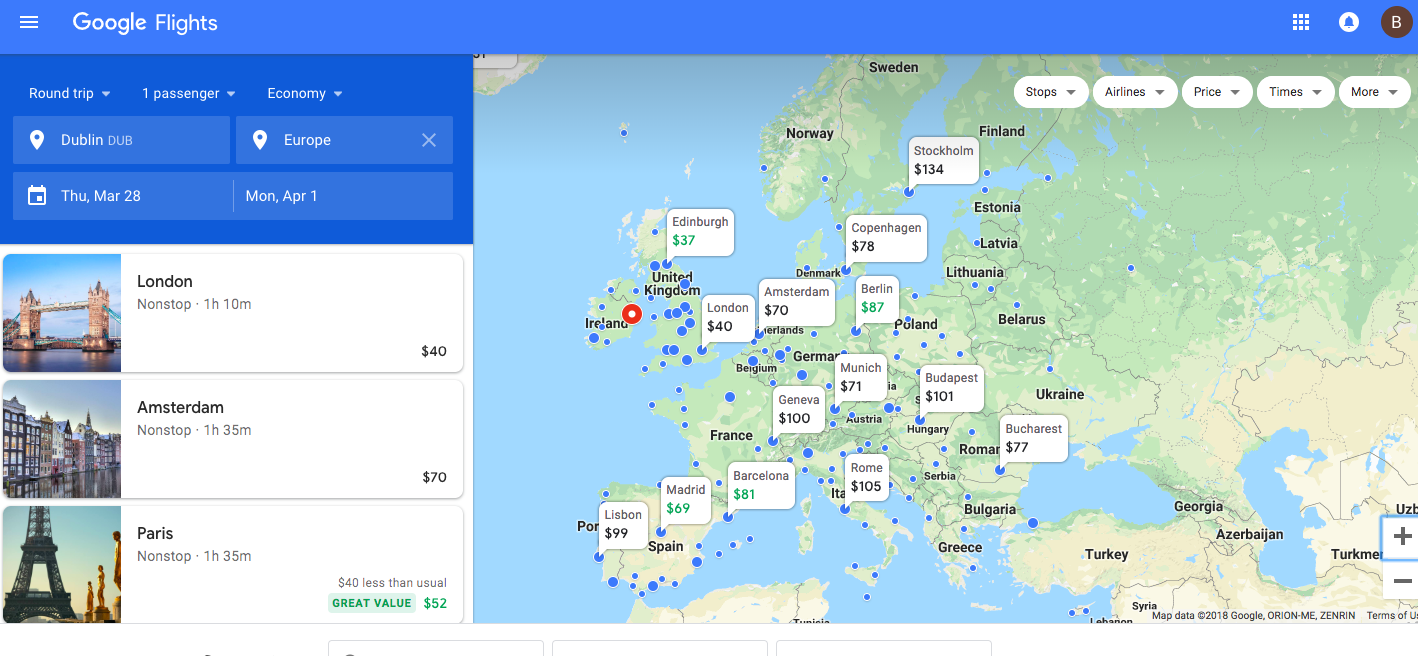The image is divided into several sections featuring different travel-related information. In the top left corner, the image includes logos of Hamco Mania, Google Flights, and a blue icon. The top right corner shows icons such as Nine Dots, a Circle, and a Bell, with a "B" embossed on the Circle.

The central portion of the image details a round-trip flight for one passenger in economy class from Dublin, Europe, departing on Thursday, March 28th, and returning on Monday, April 1st.

In the lower left section, travel options are highlighted:
- **London**: An image of the iconic London Bridge with a note of a non-stop flight lasting 1 hour and 10 minutes, priced at $40.
- **Amsterdam**: A picturesque view of numerous buildings along with a body of water and a blue sky, detailing a non-stop flight lasting 1 hour and 35 minutes, priced at $70.
- **Paris**: An image featuring the Eiffel Tower and statues with a mention of a flight costing $40 less than usual, also indicating a price of $2.

There is also a map section noted as "Bond Races map data, 2018," sourced from Google, with annotations like Ryan, B, Zen, Ryan. This map displays several European cities such as Annenberg, Stockholm, Copenhagen, Amsterdam, London, Berlin, Munich, Geneva, Barcelona, Madrid, Lisbon, Rome, Bucharest, and Budapest.

Further geographic detail includes various countries listed along the right side: Norway, Sweden, Finland, Estonia, Latvia, Lithuania, Belarus, Ukraine, Hungary, Romania, Bulgaria, Greece, Turkey, Georgia, Azerbaijan, and Turkmenistan.